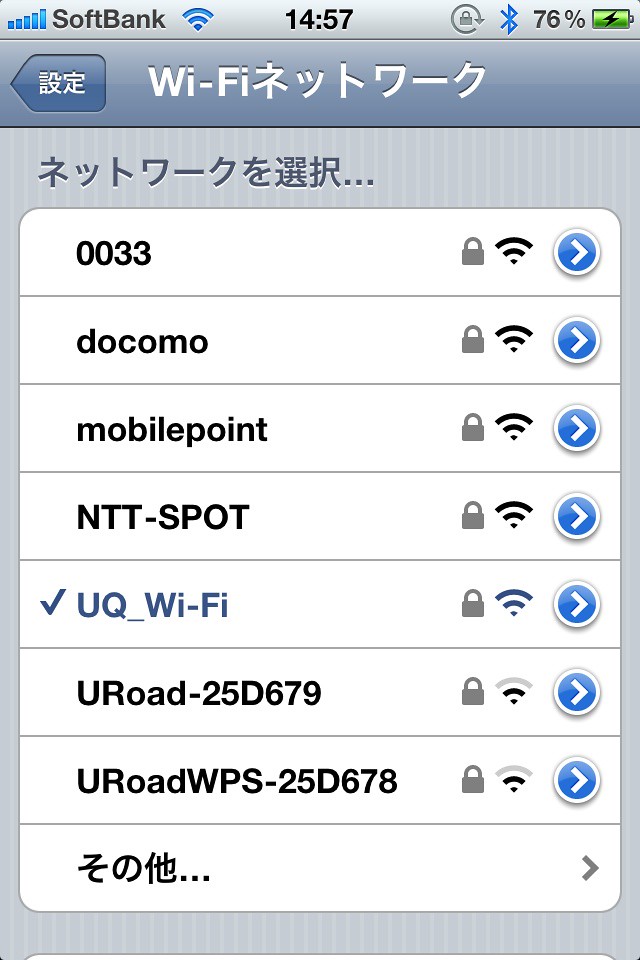This screenshot from a phone displays the Wi-Fi network selection interface, set against a light gray background. At the top, a light gray status bar shows full signal bars, "SoftBank" as the service provider, a blue Wi-Fi icon indicating connectivity, the time "14:57," and a battery icon displaying 76% in green with Bluetooth activated. Below this header, a darker gray bar features Asian characters and the text "Wi-Fi."

The main screen lists eight available Wi-Fi networks with their respective signal strengths and lock icons, indicating password protection. The networks are as follows:

1. "0033" – locked, full bars.
2. "DontDocomo" – locked, full bars.
3. "MobilePoint" – locked, full bars.
4. "NTT-Spot" – locked, full bars.
5. The connected network "UQ_Wi-Fi" – locked, full bars, with a blue checkmark.
6. "UROAD-25D679" – locked, two bars.
7. "UROADWPS-25D678" – locked, two bars.
8. A network identified by three Chinese characters, followed by an arrow – locked.

Each network entry includes the Wi-Fi symbol and a distinct blue circle with a white arrow pointing right.